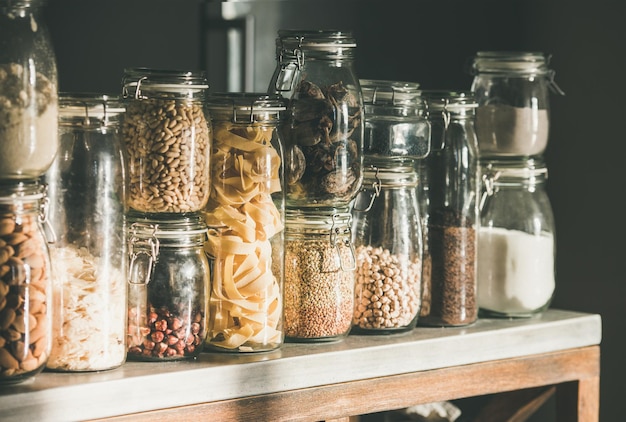The photograph captures an assortment of clear glass storage jars of varying shapes and sizes, each sealed with a rubber gasket and secured by a clamp-down wire lid. On a white or gray marble-topped table in a dimly lit kitchen, light enters from the right side, casting reflections on the jars and shadows in the background that obscure the room, although a fridge handle is faintly visible. The jars, stored both singly and in stacks of two, house a wide array of dry goods. Tall and narrow jars contain items like brown seeds and egg noodles, while shorter jars are filled with substances ranging from sugar and wheat flour to chocolate chips or nuts. Among the collection, there are also jars containing black-eyed peas, dried chili peppers, fettuccine noodles, and various kinds of beans and legumes. Some jars hold pickles, olives, and dried mushrooms, all meticulously sealed to ensure their contents are preserved. The scene evokes a sense of meticulous organization amidst a subtle play of light and shadows.